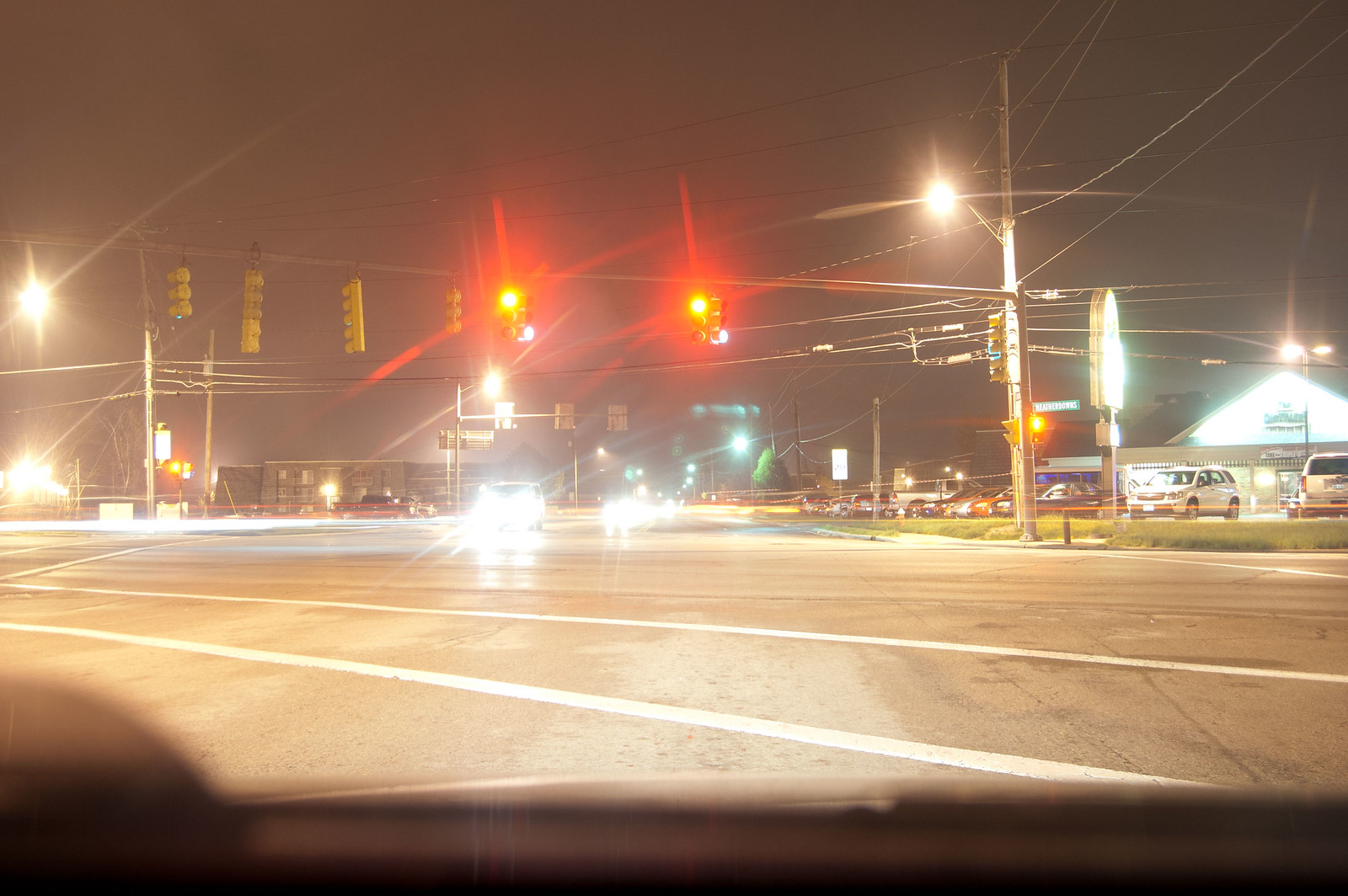A nighttime photograph taken from inside a vehicle captures an urban cityscape at an intersection. From the perspective of the driver, a small portion of the dashboard and a slight corner of the steering wheel are visible in the foreground. The vehicle is stopped at a set of two red stoplights, waiting for the signal to change. Oncoming cars, with their headlights beaming toward the driver, are also waiting at the intersection. Streetlights on the corners of the junction cast pools of light on the asphalt, illuminating the scene. Across the street, various businesses are visible, with their parking lots housing several parked cars, adding a sense of livelihood to the nighttime landscape.